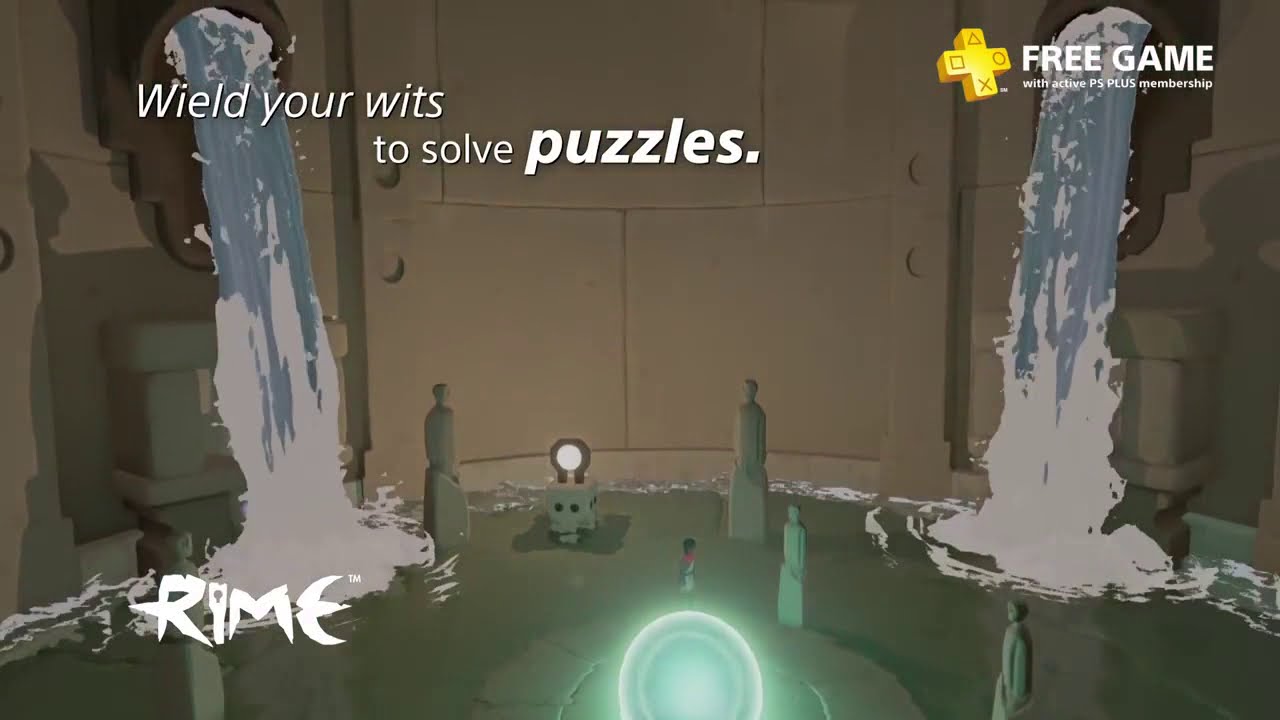The image is a detailed screenshot of a video game advertisement, showcasing a third-person perspective. The scene is set in a large, circular underground sewer treatment facility. The player character stands about 20 feet away from the camera at the far end of the cylindrical room. The floor contains a puddle of water, fed by two massive pipes approximately 30 feet up the wall, which are gushing water like waterfalls. Additionally, there are four statues resembling human figures scattered around the room, along with a glowing green orb positioned at the bottom of the graphic. In the upper right corner, there is a yellow directional pad logo for PlayStation, along with text that reads, "Free game with active PS Plus membership." In the top left corner, white text declares, "Wield your wits to solve puzzles," with the latter part of the text slightly indented to the right. The game's title, "Rime," is displayed in an old, rock-carving typeface on the bottom left corner.